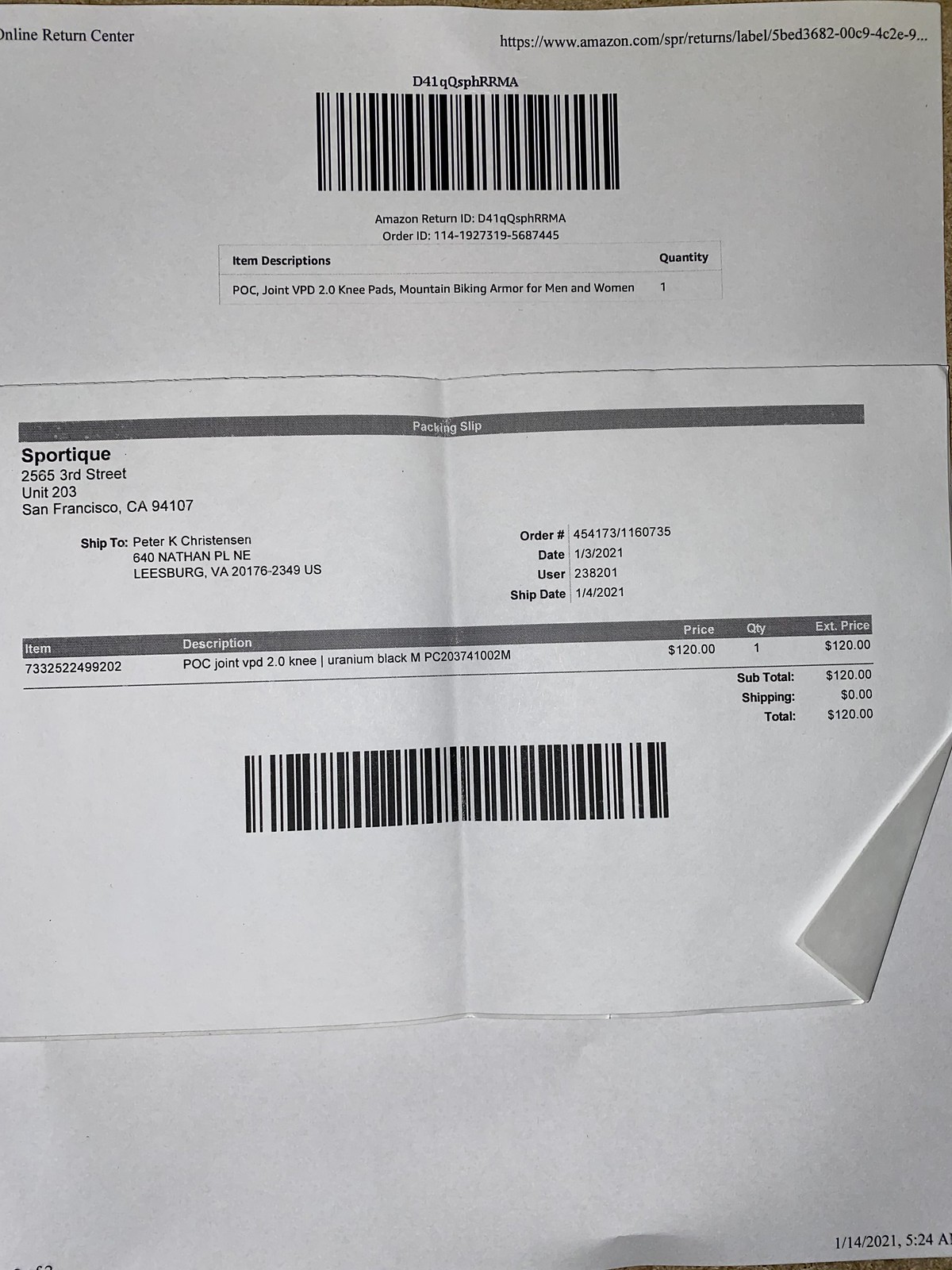The image depicts an order receipt akin to an invoice you receive after making an online purchase. The receipt, printed on a white sticker-like paper with a greaseproof background, is placed over a plain sheet of paper. At the top, the header reads "Online Return Centre" followed by a website address related to the document, indicating it is from Amazon. Below this, there is a significant barcode alongside. Further down, it lists an "Amazon Return ID" and "Order ID," each tagged with specific identification numbers. 

The item bought is described—knee pads specifically designed as mountain biking armor suitable for both men and women, and the quantity mentioned is one. The receipt provides the return destination's address, which is "Sportac" in San Francisco. Additionally, it details the shipping address: "Peter K Christensen, 640 Nathan Place NE, Leesburg, VA." The order date is noted as March 1, 2021. Completing the information, the document also includes the item’s price, listed at $120.